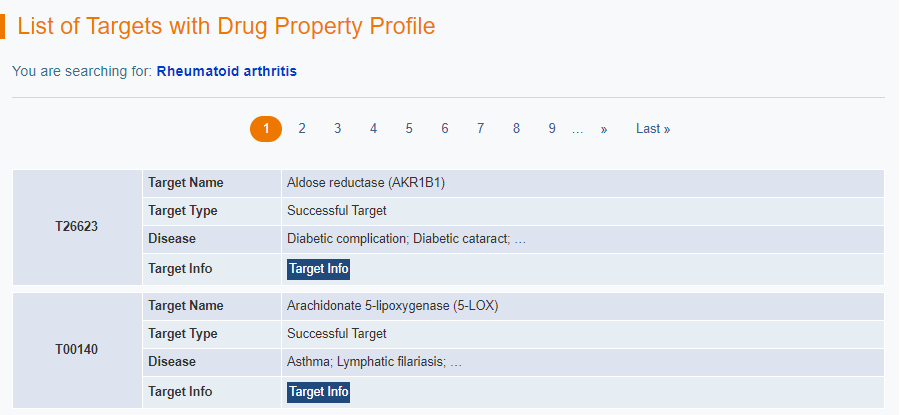Detailed Caption: 

The image shows a computer search page with a light blue background and orange text. At the top left, the heading reads "List of Targets with Drug Property Profile." The user is searching for "Rheumatoid Arthritis," which is highlighted in a darker blue.

Below this heading, a navigation bar lists numbers from one to nine, with the number one circled in orange and the others displayed in blue. To the right, two blue rectangular buttons are labeled "Arrow" and "Last" with an arrow icon beneath each.

On the left side of the page, there is a vertical list containing various data points. The sequence starts with the identifier "T26623," followed by sections labeled "Target Name," "Target Type," "Disease," and "Target Info." 

Specifically highlighted is an entry for "Aldose Reductase (AKR1B1)," marked as a successful target for diabetic complications such as diabetic cataract. The target info is represented by the code "T00140."

Further down, another highlighted entry provides details for "Arachidonate 5-Lipoxygenase (5-LOX)," indicated as a successful target for conditions like asthma and lymphatic filariasis. This entry's target info is similarly represented by a highlighted code.